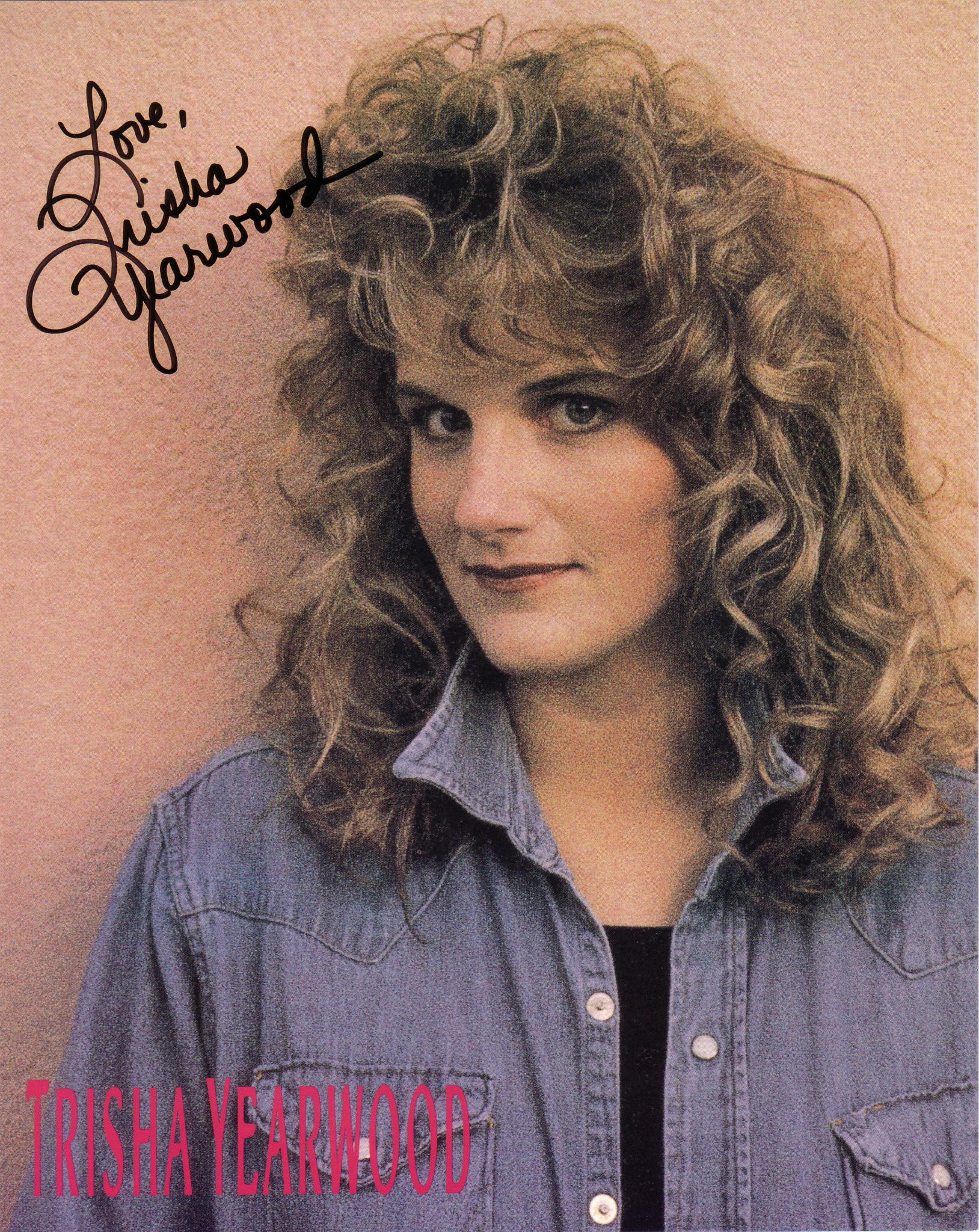This image is an autographed poster of Trisha Yearwood, the renowned country music star. The poster features Trisha Yearwood looking directly at the camera with a slight, gentle smile. She has long, curly hair reminiscent of Farrah Fawcett's style, with light brown highlights. Trisha is wearing a blue denim shirt with white buttons and chest pockets, unbuttoned to reveal a black shirt underneath. She also has dark red lipstick on. The background is a light salmon color. The top left corner of the poster bears her autograph in script, reading "Love, Trisha Yearwood," and the bottom left corner features her name in all caps, written in pink text. She is leaning against a beige wall, adding a relaxed and casual feel to the image.